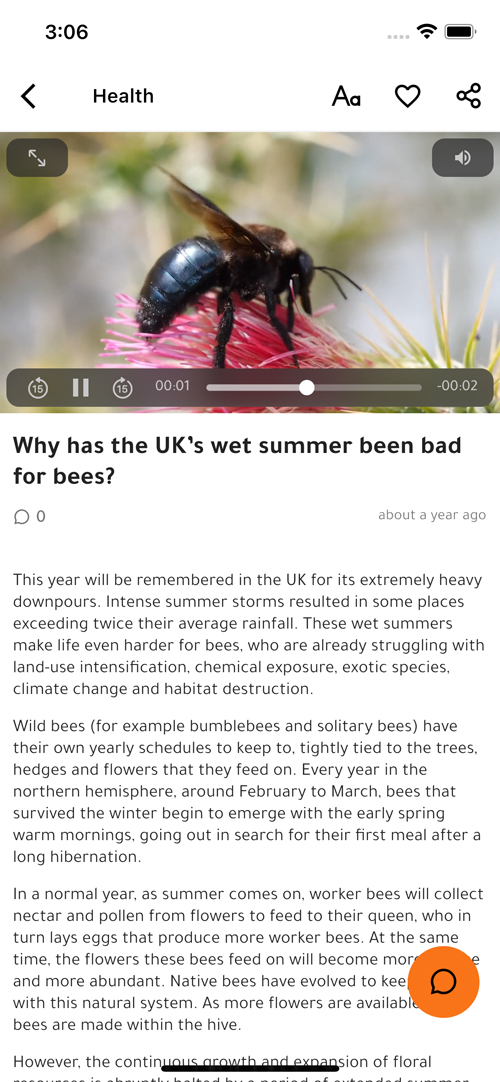The image shows an online advertisement or informational post viewed on a smartphone. The phone display, located in the top left corner, indicates the time as 3:06, alongside standard notifications, including battery status and signal strength. Dominating the center of the screen is a health-related video featuring a close-up of a black bee perched on a pink flower, set against a blurred background. This video includes controls at the bottom, such as a play button and indicators for duration and remaining time. Below the video lies a title that reads, "Why has the UK's wet summer been bad for bees?" Additionally, the post appears to include an article or detailed description on the subject, with a note stating it was posted about a year ago.